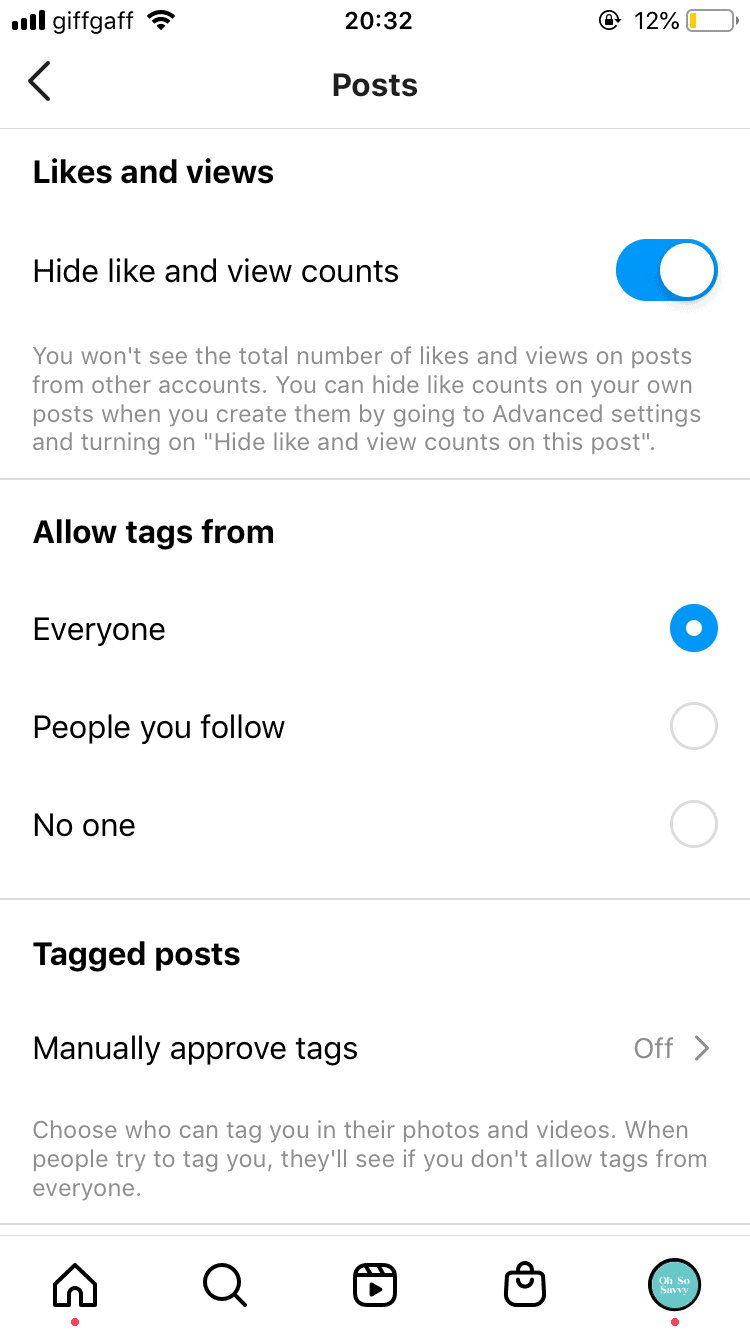This image features a detailed screenshot of Instagram's settings interface, oriented towards privacy and interaction controls.

At the very top of the screenshot, the word **'Posts'** is prominently displayed in the center, with a back button situated to its left. The first visible section is titled **'Likes and Views'**, where the toggle for **'Hide Like and View Counts'** is turned on. An explanation beneath this setting informs users that turning on this feature will prevent them from seeing the total number of likes and views on posts from other accounts. Additionally, users are advised that they can hide like counts on their own posts by navigating to **Advanced Settings** and enabling **'Hide Like and View Counts on This Post'**.

The next section, labeled **'Allow Tags From'**, presents three options. The currently selected choice is **'Everyone'**; the other options include **'People You Follow'** and **'No One'**. Further down, under the **'Tagged Posts'** section, the **'Manually Approve Tags'** option is turned off. The description accompanying this setting states, "Choose who can tag you in their photos and videos. When people try to tag you, they'll see if you don't allow tags from everyone."

At the bottom of the screenshot, the Instagram navigation bar is displayed. From left to right, this bar features the **Home** button, the **Search** button, the **Instagram Reels** button, the **Shopping Tab** button, and, on the far right side, the user’s Instagram profile picture. Notably, both the Home and Profile icons have red dots underneath them, possibly indicating notifications or recent activity.